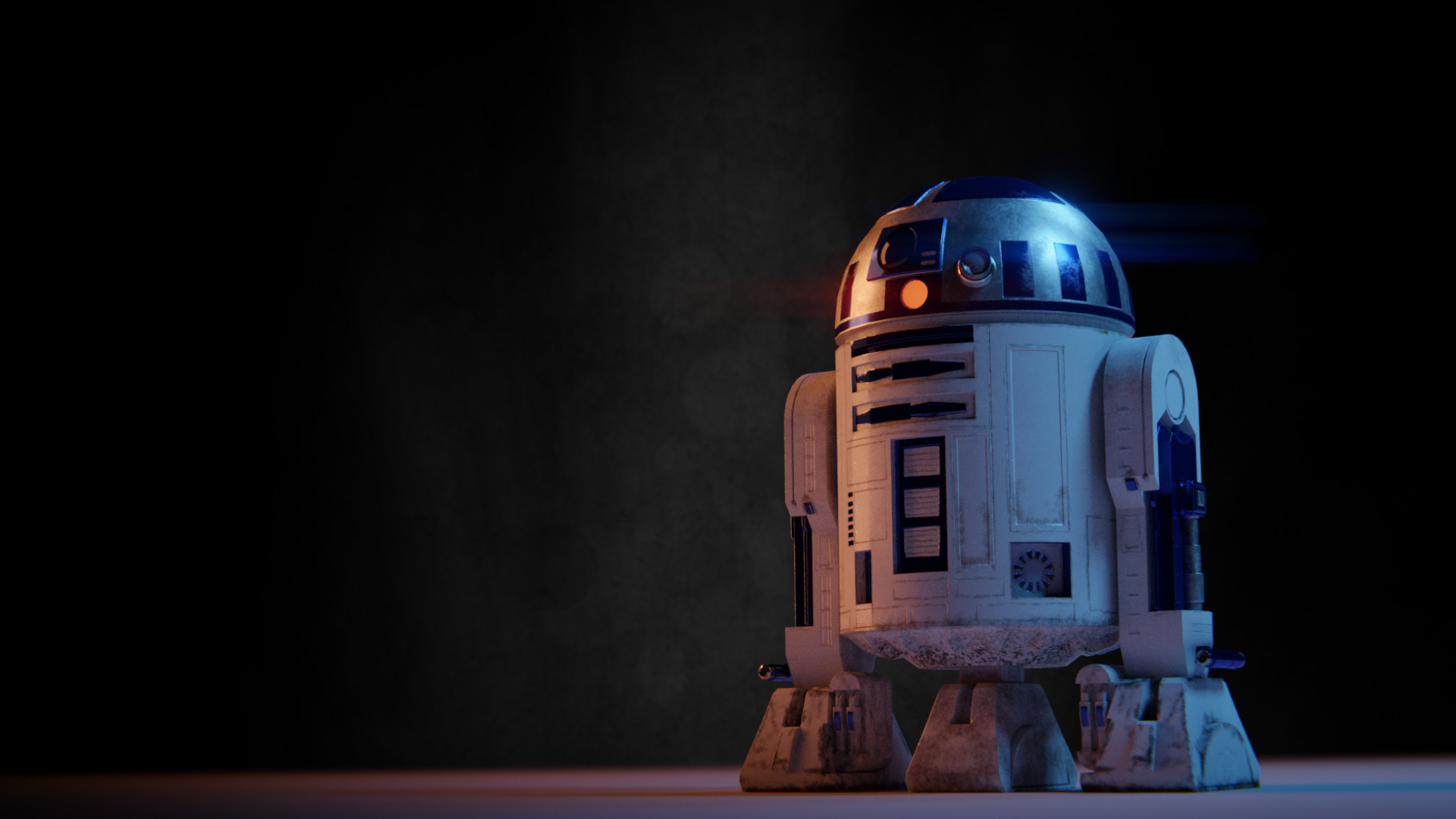This is a screenshot from the movie Star Wars featuring the iconic robot R2-D2. The image is horizontally rectangular with a dark background of black and gray tones, creating a stark contrast to highlight the robot. Positioned a few inches from the right side of the frame, R2-D2 stands with its familiar cylindrical shape and domed top. The primary color of the body is white adorned with blue markings, including several dark blue squares that light up. The dome, a bright metallic gray, carries a signature blue painted tip and various blue highlights. An orange light is prominently visible at the top of the dome, while a purple hue seems to be emanating from above. R2-D2 is supported by three legs, two on either side that curve outward into square bases and one in the center, establishing a tripod stance. The lighting cast from the left side of the image illuminates the left part of the robot more brightly, defining its contours vividly against the dark, minimalist background. Overall, the detailed depiction effectively captures R2-D2's distinctive features and ambiance in the scene.